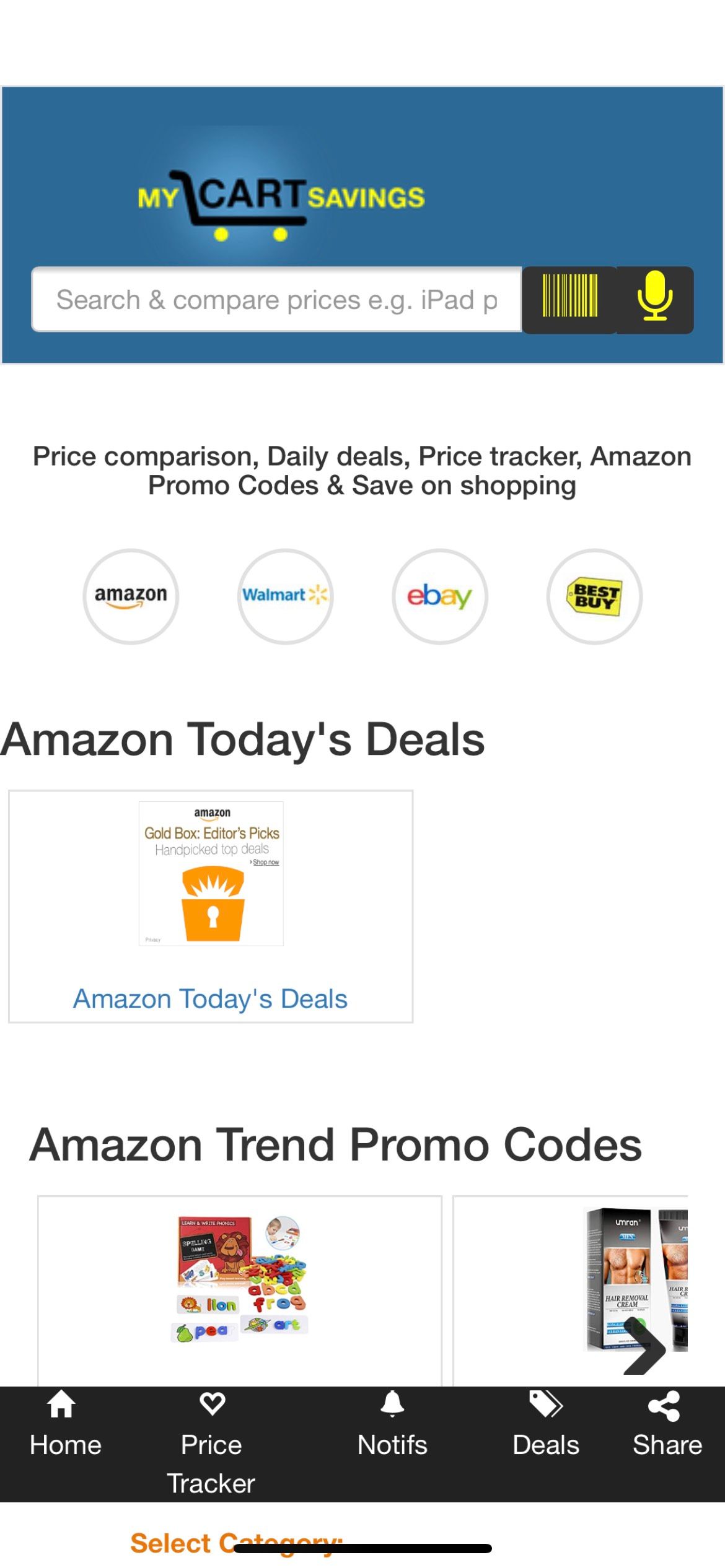This image displays a mobile website or application tailored for savvy shoppers looking to save money. The top section features a blue banner labeled "My Cart Savings," with the word "Cart" highlighted by a shopping cart icon and the words "My" and "Savings" in yellow. Directly underneath, there is a search bar with the placeholder text "Search and Compare Prices," but slightly faded is the partial text "Ichi iPad P." To the right of the search bar, a black rectangle houses a yellow barcode and a microphone icon, suggesting functionality for scanning and voice search.

The main section of the screen, occupying a white background, displays a series of options in black text: "Price Comparison," "Daily Deals," "Price Tracker," "Amazon," "Promo Codes," and "Save on Shopping." Below these options, icons representing four major online retailers—Amazon, Walmart, eBay, and Best Buy—are presented in a circular arrangement.

Further down, prominent black text announces "Amazon Today's Deals," followed by a grey-outlined box with a white interior. Inside this box, there's text reading "Amazon Gold Box Editor Picks Handpicked Top Deals" in black, accompanied by "Amazon Today's Deals" in teal further below. Another section titled "Amazon Trend Promo Codes" in large black text introduces two product images. One image seems to depict colorful alphabet magnets or stickers for children, while the other possibly shows a tube of hair removal cream for men.

At the bottom, a navigation banner features options labeled "Home," "Price Tracker," "Notifs," "Deal," and "Share," indicating essential functionalities for a comprehensive shopping experience.